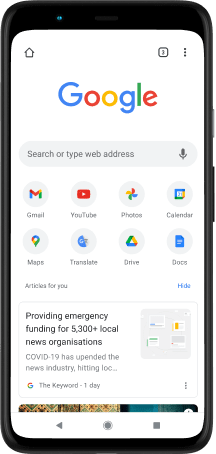## Detailed Caption of Image

The image appears to be a screenshot from a smartphone, capturing the Google homepage. The overall background of the image is a clean, crisp white. 

### Upper Section:
1. **Top Left Corner**: A faint silhouette of the front of a house is visible.
2. **Top Right Corner**: 
   - A small black box displaying the number "3."
   - To the the right of the box, there are three vertical dots arranged in a line.

### Middle Section:
1. **Google Logo**: Centrally positioned, the Google logo is displayed prominently with each letter in differing colors:
   - 'G' in blue,
   - First 'o' in red,
   - Second 'o' in yellow,
   - 'g' in blue,
   - 'l' in green,
   - 'e' in red.
2. **Search Box**: Beneath the logo, a search box is present with the text "Search or type web address" in a grayed-out color. To the far right within the search box, there is an icon of a microphone.

### Icon Section:
1. **Gmail Icon**: Represented by a multicolored "M" with sections in blue, red, green, and yellow.
2. **YouTube Icon**: Red play button symbol.
3. **Google Photos Icon**: A colorful propeller-like symbol.
4. **Calendar Icon**: Symbol of a calendar with the text "Calendar."
5. **Maps Icon**: Text "Maps."
6. **Translate Icon**: Text "Translate."
7. **Drive Icon**: Text "Drive."
8. **Docs Icon**: Text "Docs."

### Article Section:
1. **Articles for You**: Located on the left-hand side in small, grayish font.
2. **Headline Box**: Containing the following text:
   - In bold, black font: "Providing emergency funding for 5,300+ local news organizations."
   - Below this in thinner, gray font: "COVID-19 has upended the news industry, hitting LOC..." with an ellipsis indicating truncated text.
3. **Image**: To the right of the text, there is a small image with a gray background, presumably generated by a computer or AI. The image consists of four tiny pictures resembling web pages.